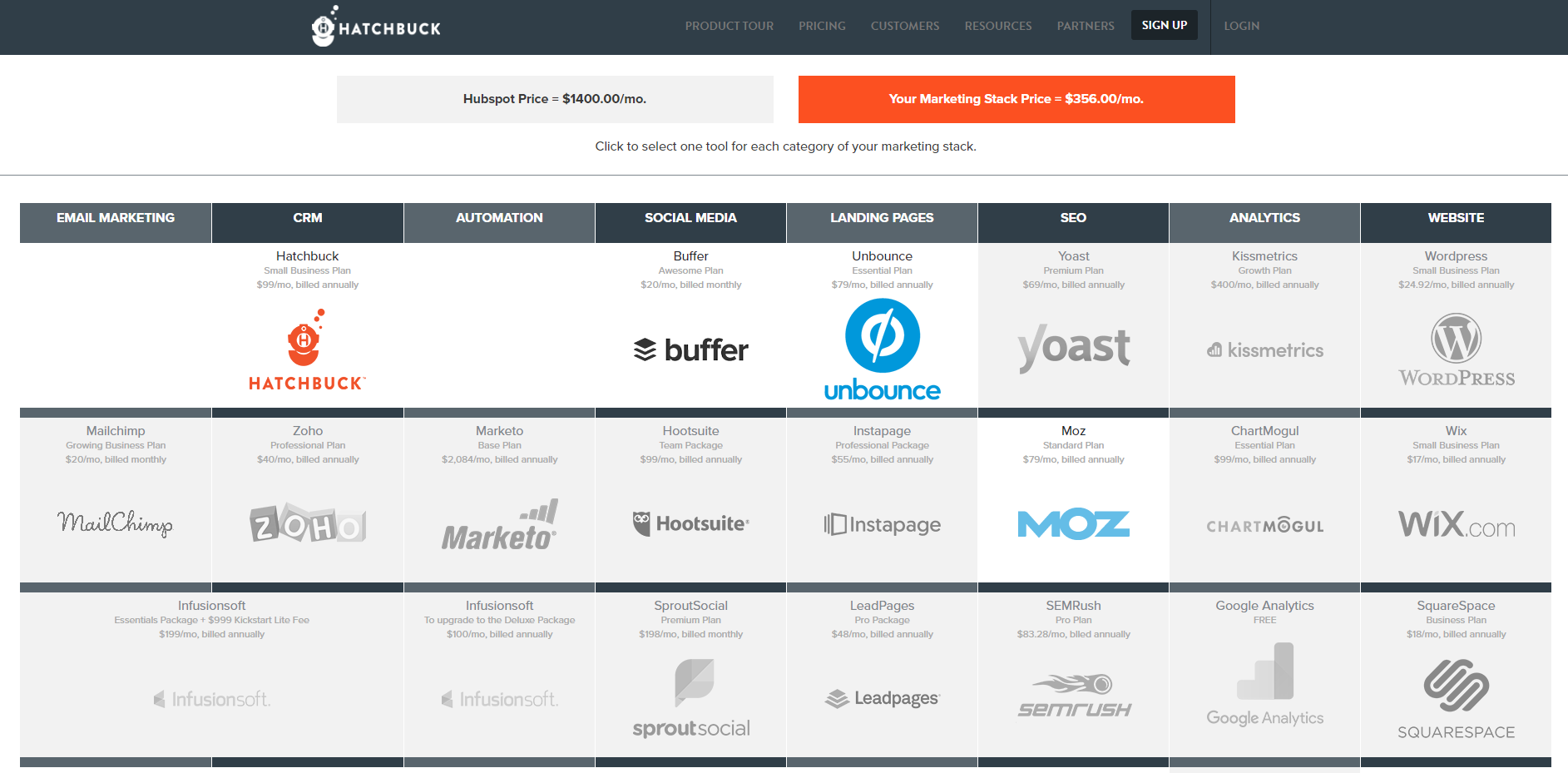Screenshot of a marketing software comparison website featuring various company logos. The page has a dark gray navigation bar at the top, displaying "Hatchbuck and Watt" on the left. To the right, there are several gray buttons labeled "Product Tour," "Pricing," "Customers," "Resources," "Earners," "Signup," and "Login." 

Directly beneath this bar, a light gray rectangular banner highlights two pricing options: "HubSpot price: $1,400 per month," accompanied by a gray button, and "Your marketing stack price: $3.56 per month," with an adjacent orange button. Below the banner, a prompt invites users to "click to select one tool for each category of your marketing stack." The main content area features a table with eight columns, showcasing an array of company logos representing various marketing tools.